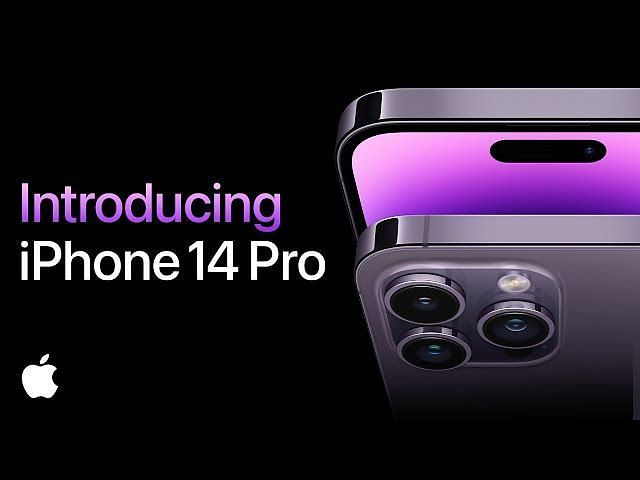The image is a rectangular advertisement depicting the introduction of the iPhone 14 Pro. At the top, the text "Introducing iPhone 14 Pro" is prominently displayed in a gradient that transitions from a light lilac to a deeper shade of lilac. Beneath the text, the white Apple logo stands out against the solid black background.

The visual design features a gradient fade effect from the visible part of the image into the black background, creating a seamless transition. The upper section of the image shows the top part of the iPhone 14 Pro, with a clear view of its camera cutout and the beveled edging of the phone. Just below this, there is another image displaying the back of the iPhone, highlighting the three individual camera lenses and the LED flash arranged within a small square module.

The solid black background enhances the clarity and prominence of the text and images, giving the advertisement a striking and modern aesthetic.